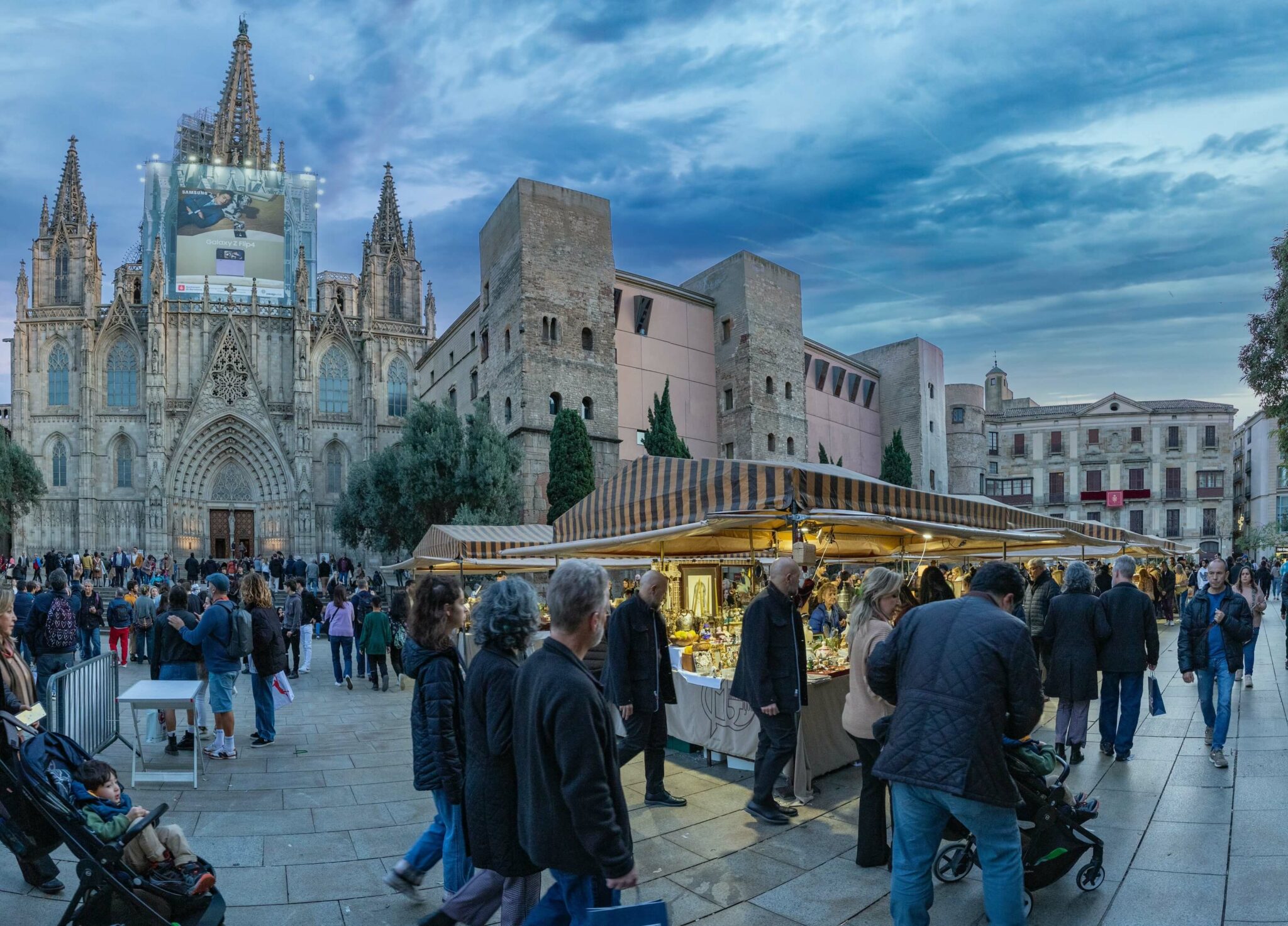In this detailed photograph, we observe a bustling central square in a European city during winter, populated by numerous tourists clad in blue and black coats and blue jeans. The left side of the frame is dominated by a large, ornate cathedral with multiple spires and arch-shaped windows, creating a dramatic architectural focal point. A considerable crowd gathers outside the cathedral, hinting at the throngs of people eager to explore its interior, which is partially visible through the open doors.

In the mid-ground, there are additional imposing buildings. One, resembling a government or municipal building with tall towers and pink stone accents between them, is partially obscured by poplar trees. Another notable structure in the foreground features stone columns and numerous windows, above which a large digital advertisement for the Samsung Galaxy Z Flip 4 is prominently displayed.

The foreground of the photograph is animated by rows of identical market stalls adorned with ivory and maroon roofs, where vendors sell various small items. This marketplace is teeming with shoppers, many of whom carry bags and some push strollers, including a woman with a toddler in the bottom-left corner of the image. The overall scene exudes the vibrant energy of a popular tourist destination on an overcast, early evening.